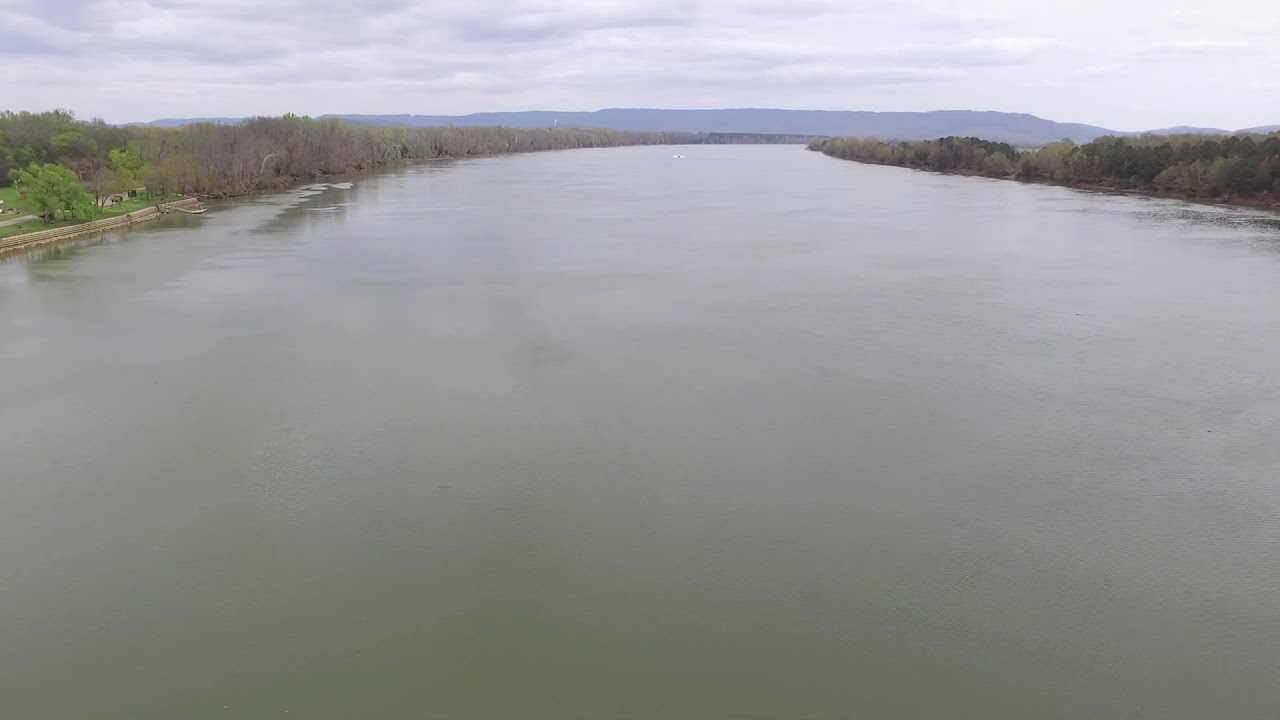A vast, smooth river dominates the scene, stretching from the bottom of the image and veering towards the right as it flows upward. The water, characterized by a murky green hue, reflects the hazy and cloud-filled sky above, although the reflection is somewhat blurry. The riverbanks are densely lined with trees; the left bank is a mix of verdant green trees and stark, leafless ones in shades of dark gray and brown, while the right bank features predominantly dark green foliage with a few lighter leaves interspersed. In the distance, a ridge of flat-topped mountains appears bluish due to their atmospheric perspective. A white barrier marks the point where the river water kisses the left bank, near which stands a house with white walls and a brown roof, fronted by a green lawn. The right bank's tree line is thick and lush, contributing to the feeling of a dense, forested area. Tying the natural elements together, a subtle pathway or nature trail can be glimpsed, inviting viewers to imagine a leisurely walk through this serene and slightly overcast landscape.